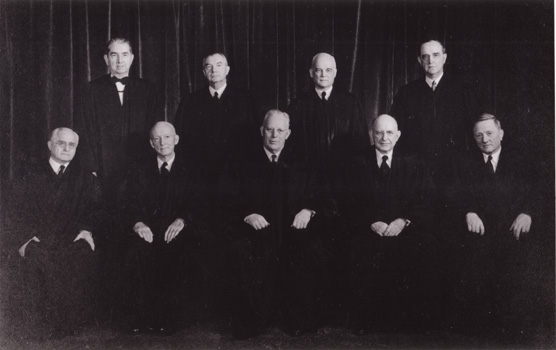This black-and-white image depicts nine elderly, white gentlemen who appear to be judges or officials, potentially older Supreme Court justices. The group is arranged with five men seated in the front row, their hands resting on their laps, while four men stand behind them, between each of the seated figures. All are clad in dark black robes over white collared shirts and ties, except for the man on the upper right who is distinctively wearing a bow tie. Although the photo itself is dark, the heads, upper sections of their robes, and possibly some hands are visible. The backdrop consists of a curtained wall, adding to the professional setting of the image. The men radiate a solemn professionalism, with reserved expressions that suggest gravity and importance, rather than overt happiness.